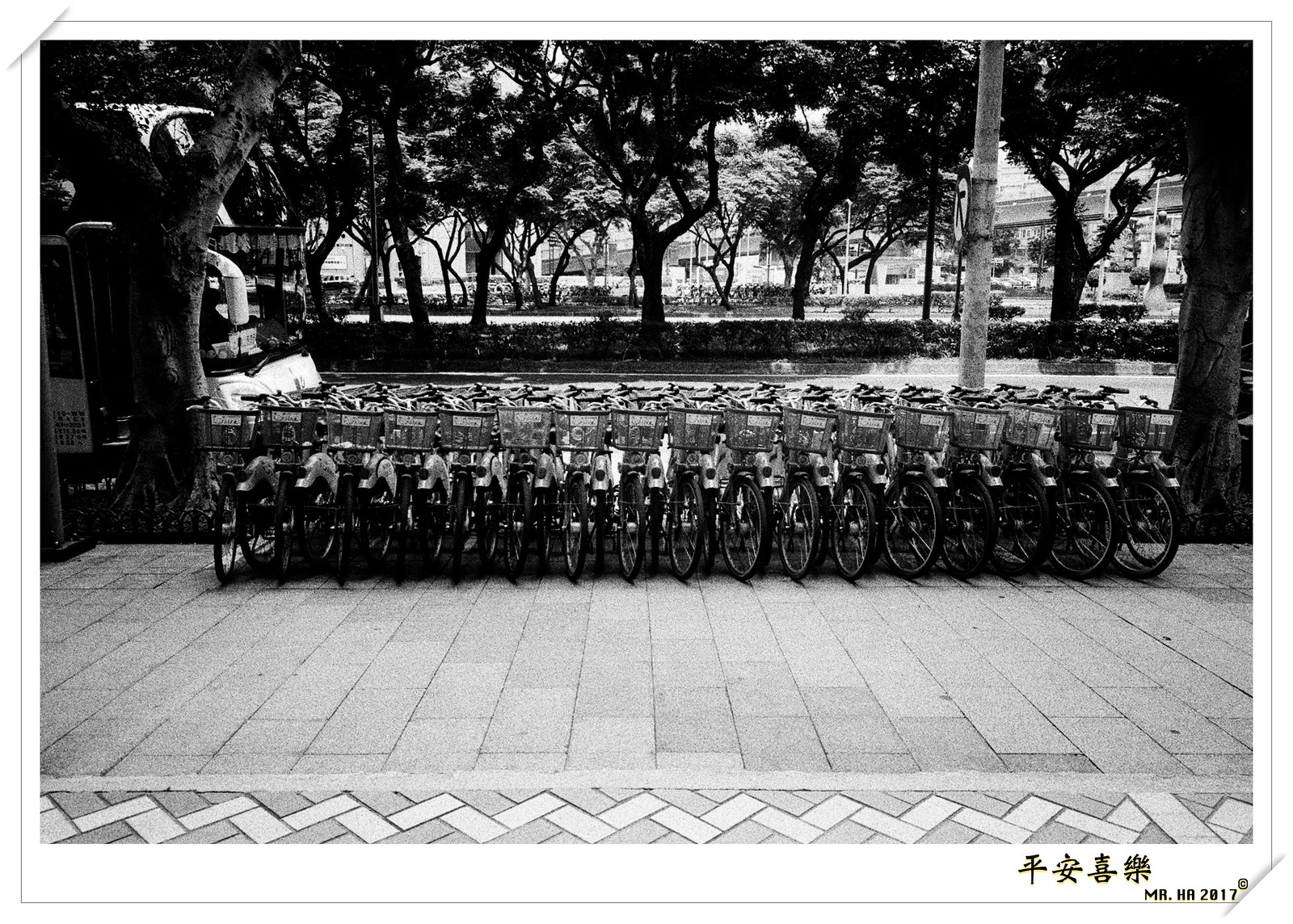This professional black and white photograph, bordered in white with a gold signature at the bottom right reading "Mr. Ha 2017" beneath several Chinese characters, captures a meticulously arranged row of approximately 20 bicycles. Each bicycle, identical in appearance and featuring a metal basket with an unreadable white placard, faces the viewer head-on. They are neatly aligned on a tiled sidewalk, interspersed with both light and slightly darker-colored bricks, stretching from the left to the right of the image. Flanking the scene are two large trees, one on each side. In the background, a garden enclosed by a wall is visible, along with additional trees and a street sign indicating no right turn. A bus can be seen on the far left, reinforcing the urban environment depicted. The overall composition, lacking any people, emphasizes the uniformity and orderliness of the bikes against the structured backdrop.